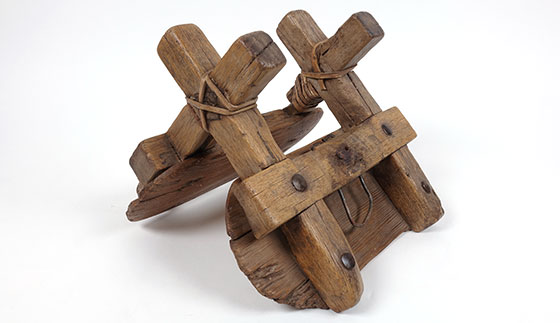This image shows an antique wooden pack saddle, meticulously crafted and aged. The structure features two solid slabs of wood at the bottom, joined at nearly a 90-degree angle. Rivets secure additional wooden pieces that rise and converge at the top, each side forming a cross. A horizontal piece of wood, located just above the bottom slabs, is held by a rust-colored rivet. Below this horizontal piece lies a U-shaped, rusted wire. The crosses on either side are reinforced by brown leather strings, tied in an X pattern. One of these strings is notably wrapped more securely around one side of a cross. The saddle is positioned at a slight angle, facing slightly to the right and toward the viewer, casting a subtle shadow on the white background. The entire piece exhibits the wear and craftsmanship of a carefully constructed, vintage item.